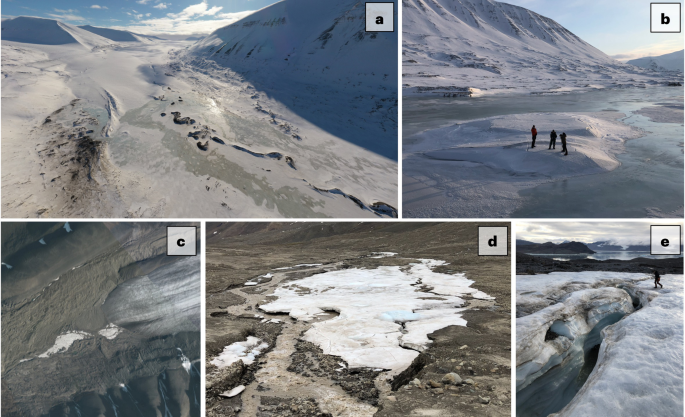A collage of five photographic images labeled A through E showcases diverse glacial and arid landscapes. In image A, there is a desolate tundra with dark grey hillsides and a clear blue sky, where the middle area is predominantly covered in white and brown snow. Image B features three people in winter gear standing on white snow or ice in a valley surrounded by grey mountain tops, with a glacier visible on the far left. Image C presents a view with brownish, greyish, and silver hues, likely depicting a glacier. In image D, a patch of white snow contrasts with the arid, rocky plain encircling it. Finally, image E captures a person navigating through a glacier-like terrain with visible cracks in the snow, set against a backdrop of mountains and a nearby lake.